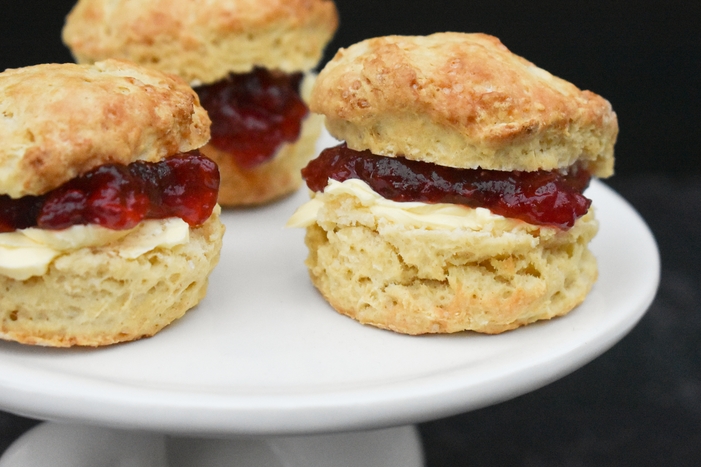The image is a highly detailed color photograph taken in a horizontal orientation, likely by a professional food photographer. It depicts a white ceramic cake stand set against a solid black background, ensuring the focus remains entirely on the food. Atop the stand, three golden-brown scones are arranged. Each scone is sliced open and generously filled with a thick layer of clotted cream at the bottom, topped with a rich, red jam, possibly strawberry or raspberry. The jam in the scone at the back appears so abundant that it looks like it might spill over the edge. The white plate and the slightly blurred base of the stand add texture and depth to the image, enhancing the visual appeal of the perfectly baked, delicious-looking scones.